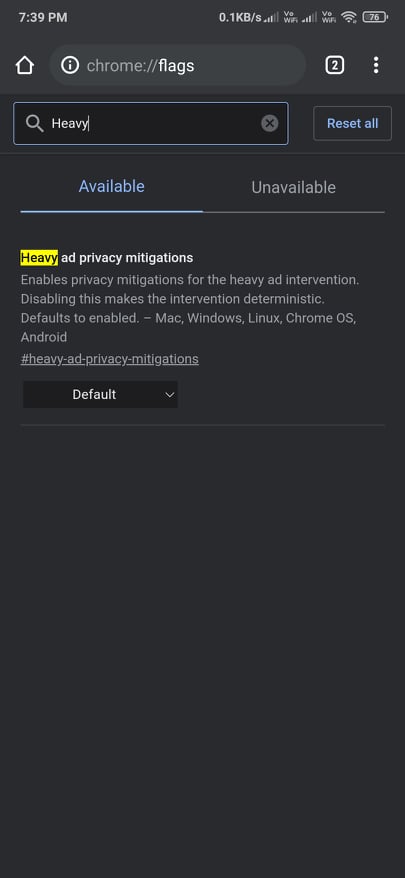A screenshot captured at 7:39 p.m. with a file size of 0.1 Kbyte/s displays the top system bar, showing icons for signal strength, Wi-Fi, and a battery percentage at approximately 76%. 

The image has a gray background with a combination of white and blue text. Below the system bar, there is a white house icon next to a white circle with an 'i' in it. The text reads, "chrome://flags". 

Further down, there's a box containing the number two and three vertical white dots. A black search box with a white magnifying glass icon and white text is present, along with a gray 'X' and a blue 'Reset all' box.

Two sections labeled 'Available' and 'Unavailable' are shown, with 'Available' highlighted in blue and 'Unavailable' in gray. The focus is on a feature option: the "Heavy Ad Privacy Mitigations."

Highlighted in gold, the description reads:

"Heady Ad Privacy Mitigations: Enables privacy mitigations for the heavy ad intervention. Disabling this makes the intervention deterministic. Defaults to enabled. Mac, Windows, Linux, Chrome OS, Android. #heavy-ad-privacy-mitigations".

Next to the description, there's a black and white dropdown menu set to 'Default' with a small arrow indicating expandability.

Below this, a thin gray line separates the content, leading to a large, blank black box with no text. The font used throughout is noted to be easy to read and visually impaired friendly.